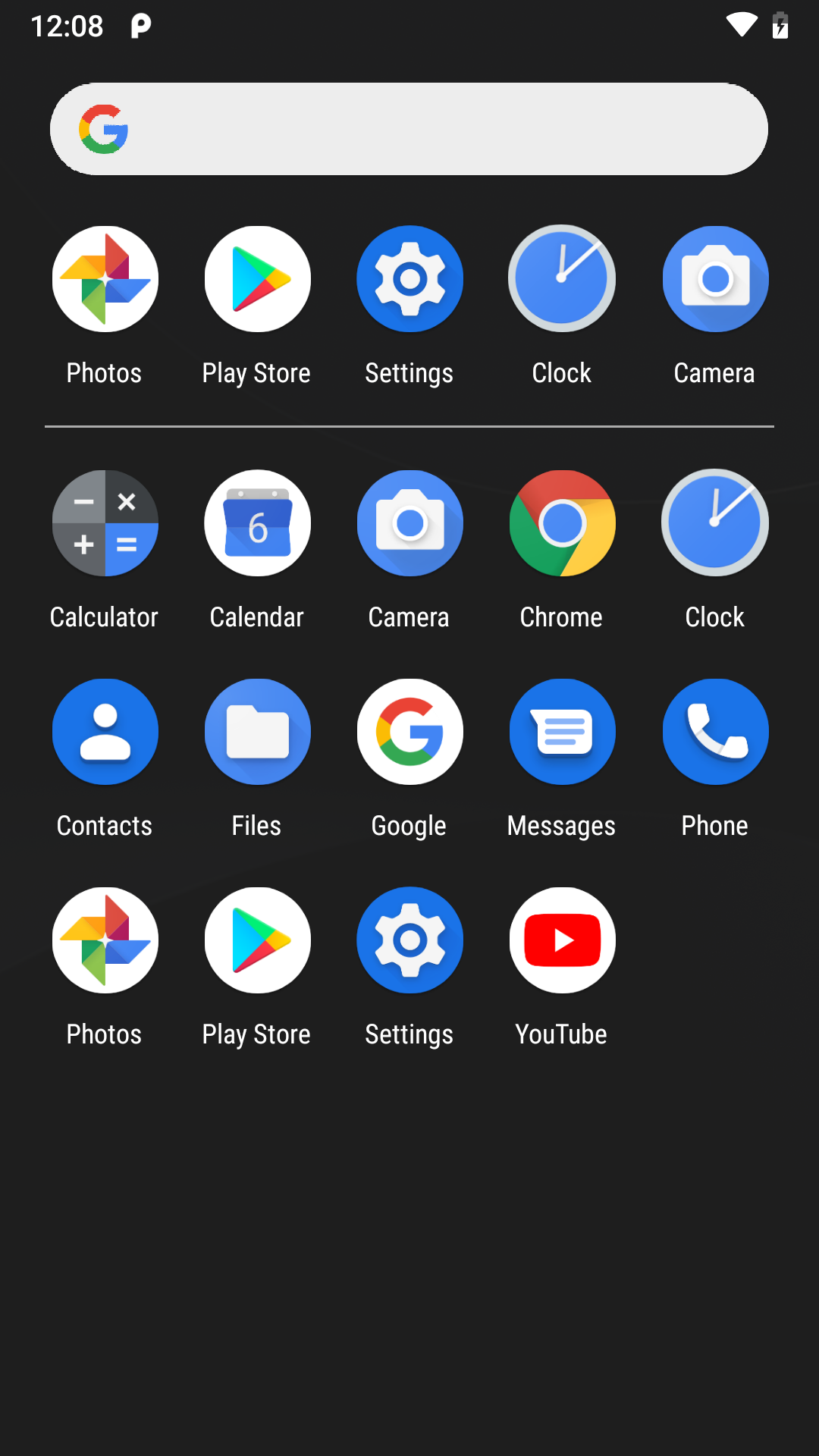The screenshot depicts a cell phone's homepage with various elements visible. 

In the upper left-hand corner, the time "12:08" is displayed in white font. To the right, there is a white "P" icon, potentially for PayPal. Moving further right, the status bar shows a half-filled battery icon with a black lightning bolt, indicating the device is charging, alongside a fully filled Wi-Fi indicator. 

Below the status bar, a white search bar with the Google "G" logo—featuring its signature red, yellow, green, and blue colors—is prominently displayed.

The app layout begins with a row of five favorite icons, separated by a thin white line from the rest of the apps. This favorite row includes Google Photos, Play Store, Settings, Clock, and Camera.

Below the favorites, the apps are organized into three rows:
- First row: Calculator, Calendar, Camera, Chrome, and Clock.
- Second row: Contacts, Files, Google, Messages, and Phone.
- Third row: Photos, Play Store, Settings, and YouTube.

Each app is represented by its distinctive icon for quick identification. The entire interface is set against a sleek, black-colored wallpaper, giving the home page a minimalist and modern aesthetic.